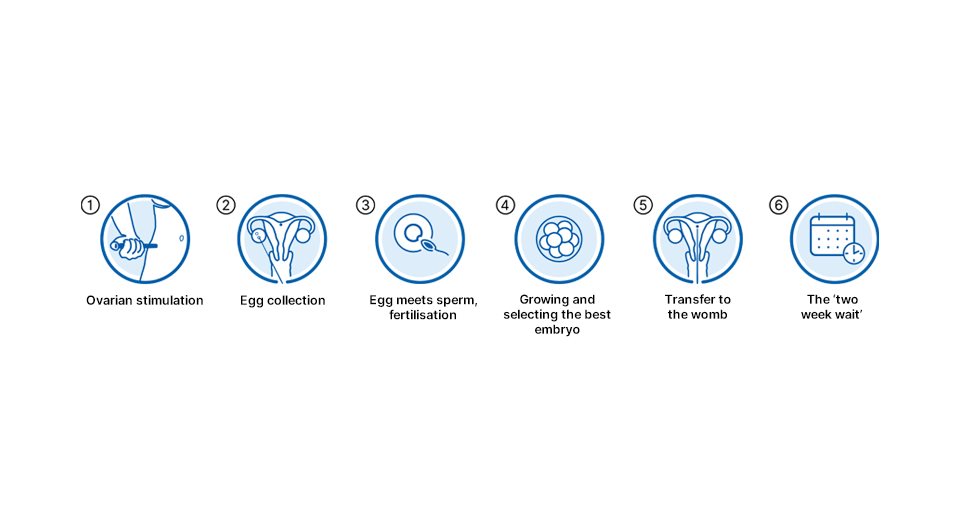The image features a detailed diagram set against a white background, showcasing a six-step process related to early stages of pregnancy. The diagram consists of six dark blue circles, each containing blue and white drawings that illustrate different steps in the process. These circles are arranged side by side, running from left to right, and each is marked in the top left corner with a small black circle containing numbers 1 to 6.

Below these images, there is descriptive black text that labels each step: "Ovarian Stimulation," "Egg Collection," "Egg Meets Sperm Fertilization," "Growing and Selecting the Best Embryo," "Transfer to Womb," and "The Two-Week Wait." The illustrations within the circles depict various aspects of a woman's body relevant to each step, including representations of a uterus and medical tools. The final circle also includes imagery of a calendar and a clock, indicating the wait period. This comprehensive depiction serves as a visual guide to the initial stages of pregnancy, from ovarian stimulation through to the waiting period post-embryo transfer.